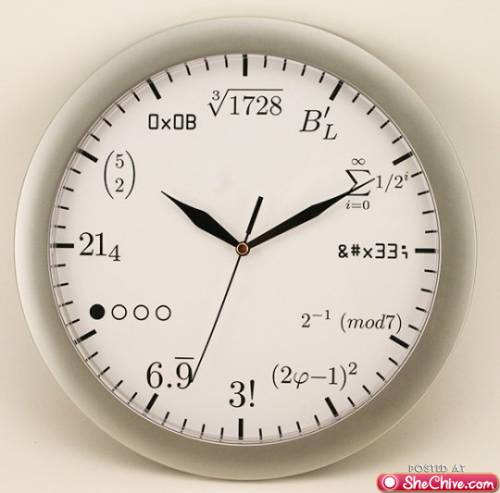This is an internet image of an unusual wall clock displayed on a clean, white background. The image bears a watermark at the bottom right corner with the text "posted at thechive.com" written in white letters on a red, semi-circular banner that includes a small white dot outlined in white. The clock has a metallic grey frame and features a unique design where traditional numerals are replaced with various mathematical equations that resolve to the corresponding numbers. The clock's face is white, and its hands are set to a time just after 10:10 and 34 seconds. Each hour mark comprises different mathematical notations, such as a cube root at 12 o'clock, factorial notation at 6 o'clock (represented by three exclamation points), and a visual representation involving circles at 8 o'clock. The minute markers are indicated by small dashes, with heavier dashes marking every five minutes. This convergence of art and mathematics makes the clock not only a functional time-teller but also a whimsical intellectual challenge.